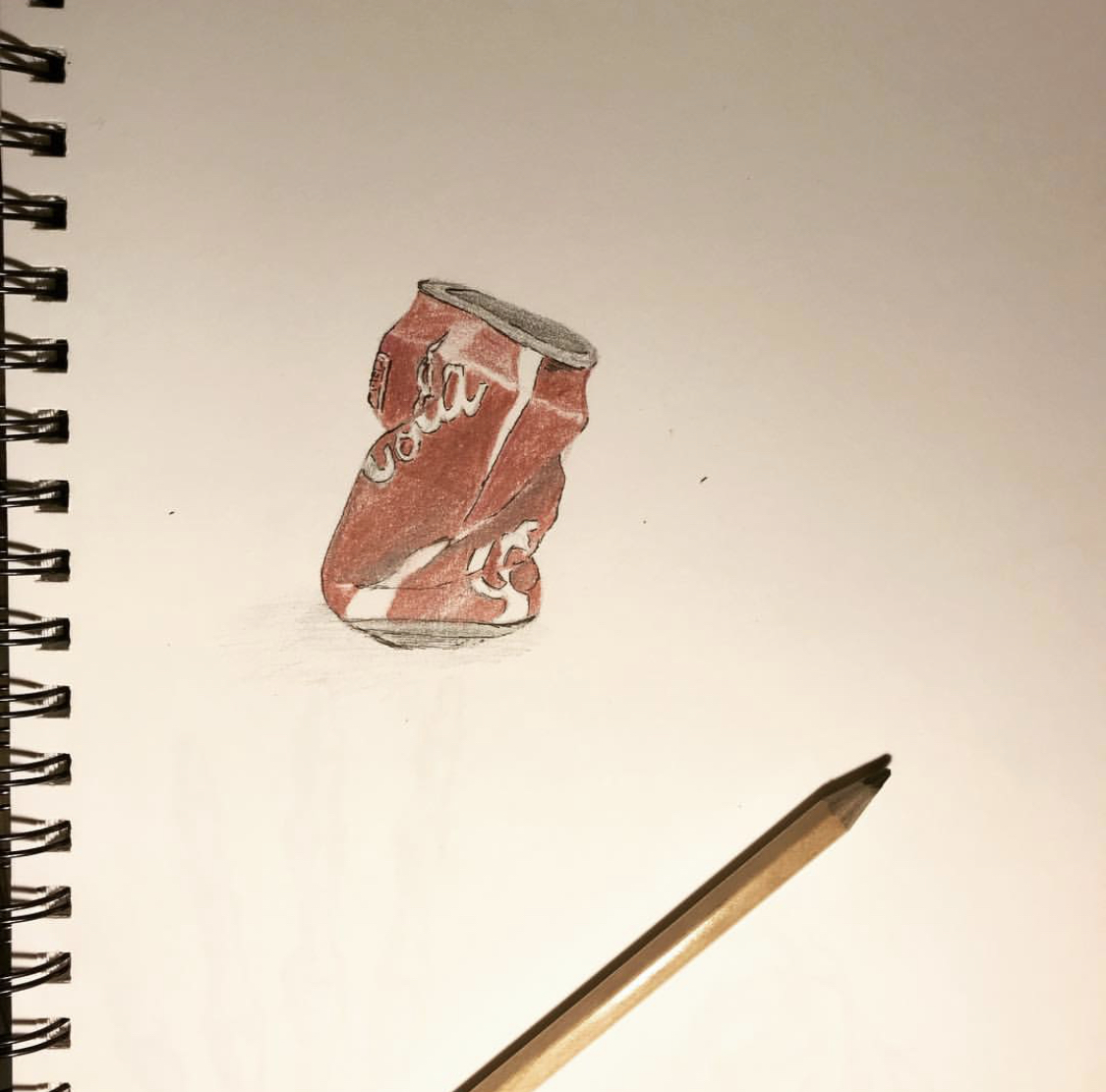In this detailed illustration, a piece of paper from a spiral notebook, most likely a drawing pad, takes center stage. The silver spirals thread through square-shaped perforations along the left edge of the paper. A sharpened yellow pencil, showing its graphite tip, lies diagonally across the bottom middle of the page, casting a subtle shadow.

Above the pencil, the artist has skillfully drawn a crushed Coca-Cola can in vivid detail. The can appears to have been compressed by hands twisting at both the top and bottom, creating creases and folds that add depth and realism to the sketch. Despite the deformation, the iconic Coca-Cola branding remains recognizable, with the letters "C-O-L-A" partially visible in white. Accentuating the creases are fine white lines, enhancing the texture of the can's surface. The top of the can is rendered in metallic hues, while the body, true to its original design, is a vibrant red. The drawing captures the essence of the crushed can, evoking a sense of realism and tactile experience.